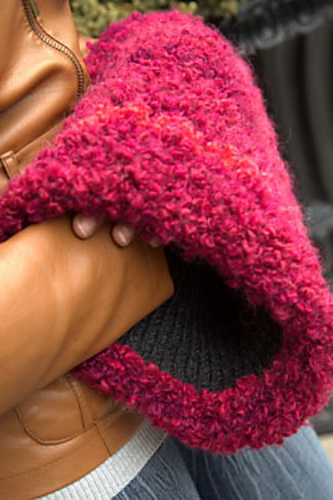The image depicts a close-up of an individual, most likely a woman, wearing a light brown leather jacket with a gold zipper. Her fingers, showing a French tip manicure, peek out from a large maroon arm warmer that appears handmade. This accessory, which has a knit black interior and a woolen exterior, envelops both her hands with her middle, ring, and pinky fingers visible at one end. Beneath the jacket, she wears a thermal shirt, and the bottom part of the image hints at a gray skirt or tights. The background features a bokeh effect with green plants and a black curtain or fence, suggesting an outdoor setting.